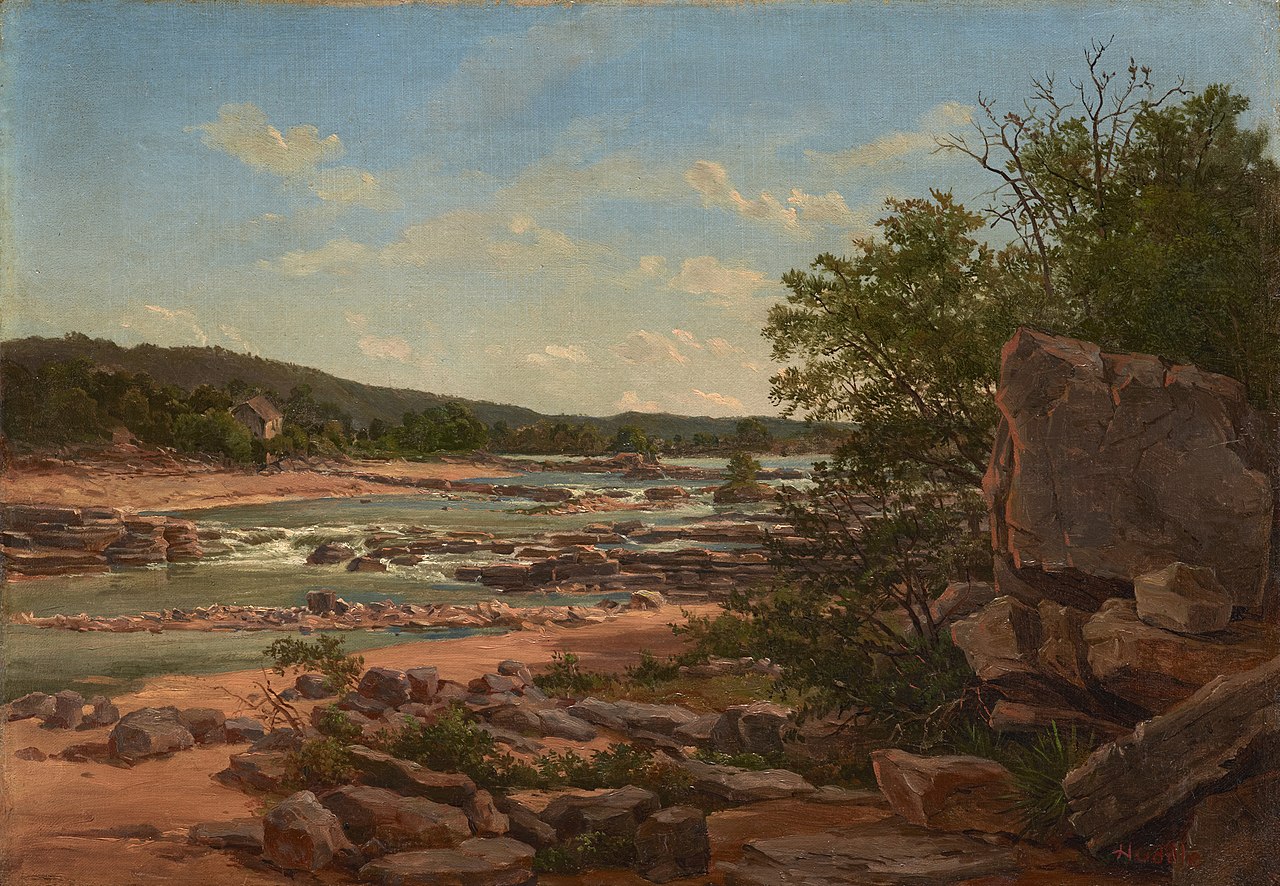This horizontal rectangular image captures a vivid and detailed landscape scene. At the forefront, there's a shoreline defined by craggy, red-colored rock formations emerging from a reddish-brown, clay-like ground. Adjacent to these rocks, green bushes sprout vibrantly. The water, possibly a river or creek, flows through these rocks with a brownish-green hue, creating white foam as it cascades over the uneven terrain, resembling gentle rapids. To the left, there’s a rocky hillside covered with additional bushy greenery, and in the distance on the opposite bank, trees and what appears to be a small house can be observed, backed by a small hill or mountain. The sky overhead transitions from a deeper blue at the top to lighter shades as it nears the horizon, punctuated by fluffy white clouds. Overall, the painting evokes the richness and serenity of a rocky riverside landscape.